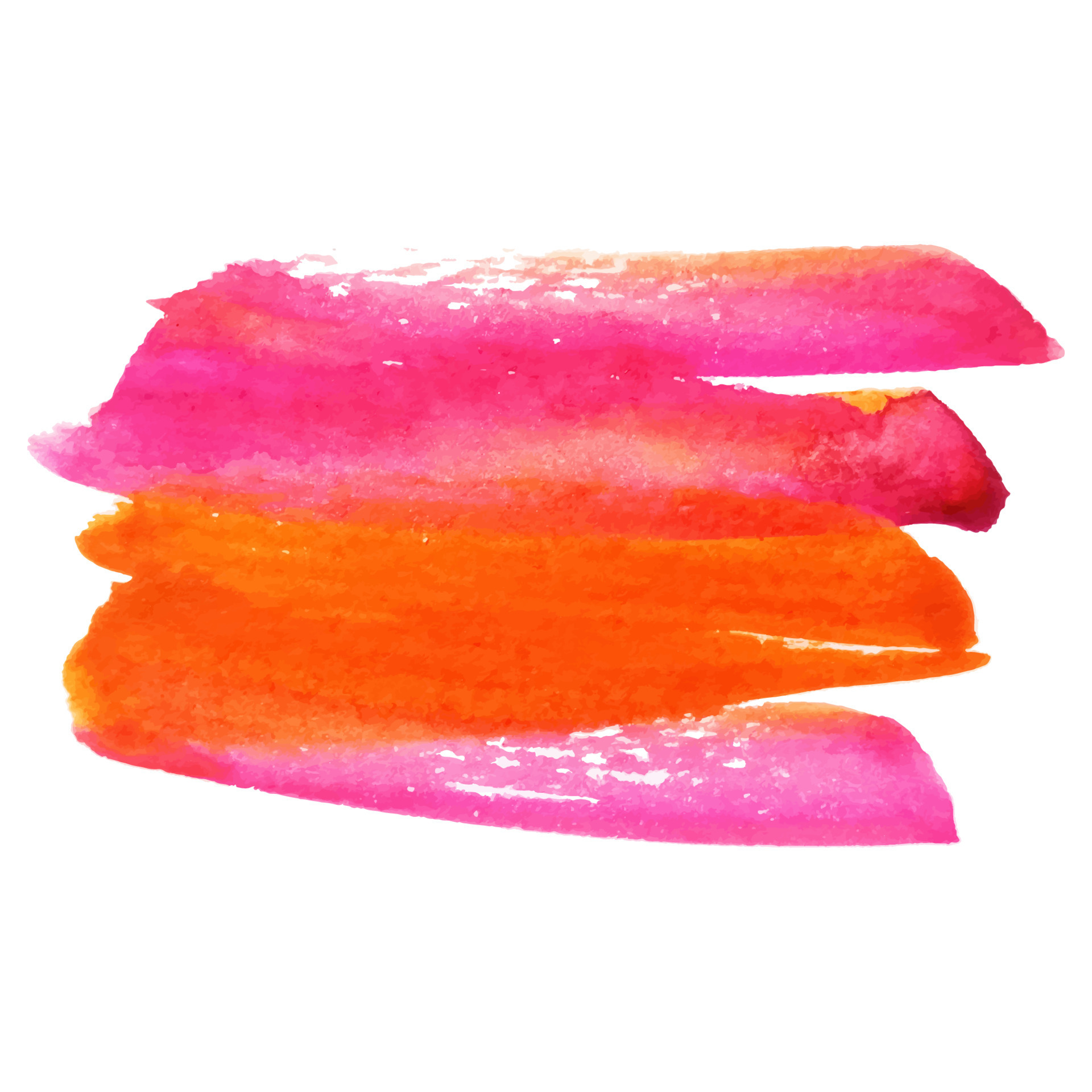The image features a minimalistic artwork with a clean, white background showcasing a series of horizontal brush strokes. There are five distinct strokes that appear to have been created with a small paintbrush, possibly using watercolor or a similar medium. Starting from the top, the first stroke is a light pink with some sections appearing faint, allowing white from the background to show through slightly. Beneath it, a darker pink stroke contains hints of orange. The third stroke is a vibrant orange, wider than the others, followed by another pink stroke tinged with orange, angled slightly downwards. The bottom stroke is a darker pink with more pronounced orange tones. Collectively, these strokes vary slightly in width, beginning wider on the left and narrowing to a point on the right, each with a delicate texture that suggests they might have been created by someone cleaning their brush. The overall composition is simple yet visually engaging, with subtle color gradations and a sense of casual, spontaneous movement.